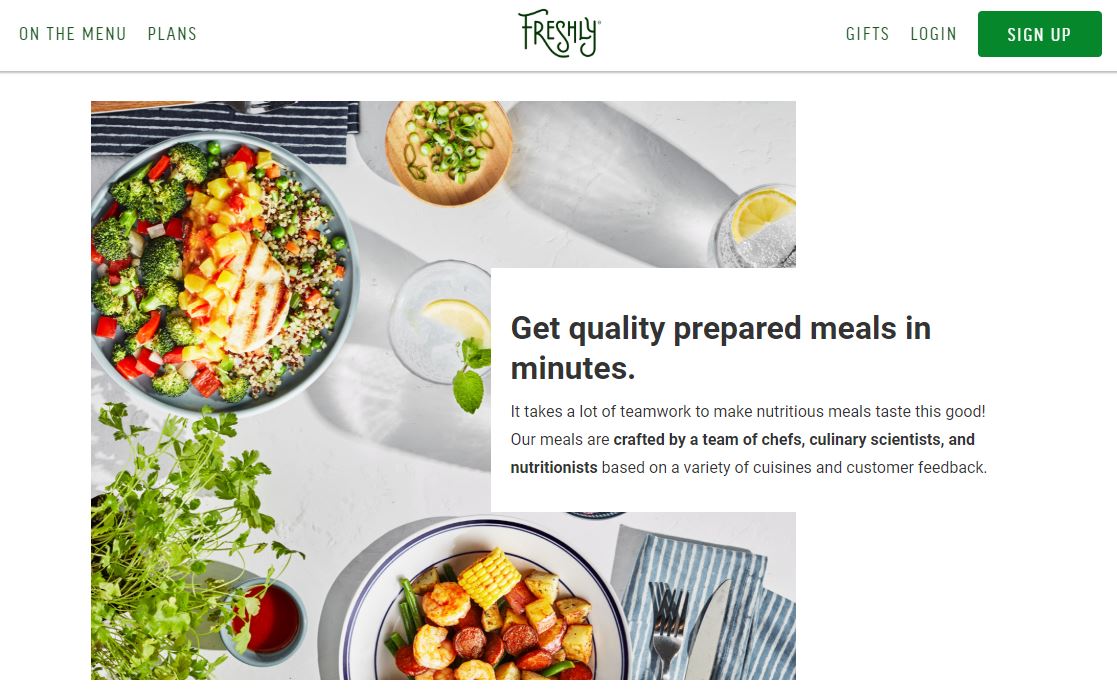The front page of the Freshly website captures a clean, organized layout designed to attract customers to this meal delivery service. At the top of the page, a horizontal menu bar extends across a white background. This header features green font with navigational options including "On the Menu" and "Plans." The company's logo, "Freshly," is prominently displayed in the center of this bar. To the right, users can find options labeled "Gifts," "Log In," and "Sign Up."

Below this header, the main section of the webpage showcases appetizing images of the food offered by Freshly. These food items are elegantly arranged on a table, each served on stylish plates. The table setting also includes appealing greenery and decorative touches, such as blue and white napkins and polished silverware. One dish prominently features an array of fresh vegetables, while another plate displays a vibrant mix of rice or couscous, also complemented by fresh vegetables. Adding to the visual appeal, a couple of glasses on the table cast interesting shadows, enhancing the overall aesthetic of the dining experience depicted.